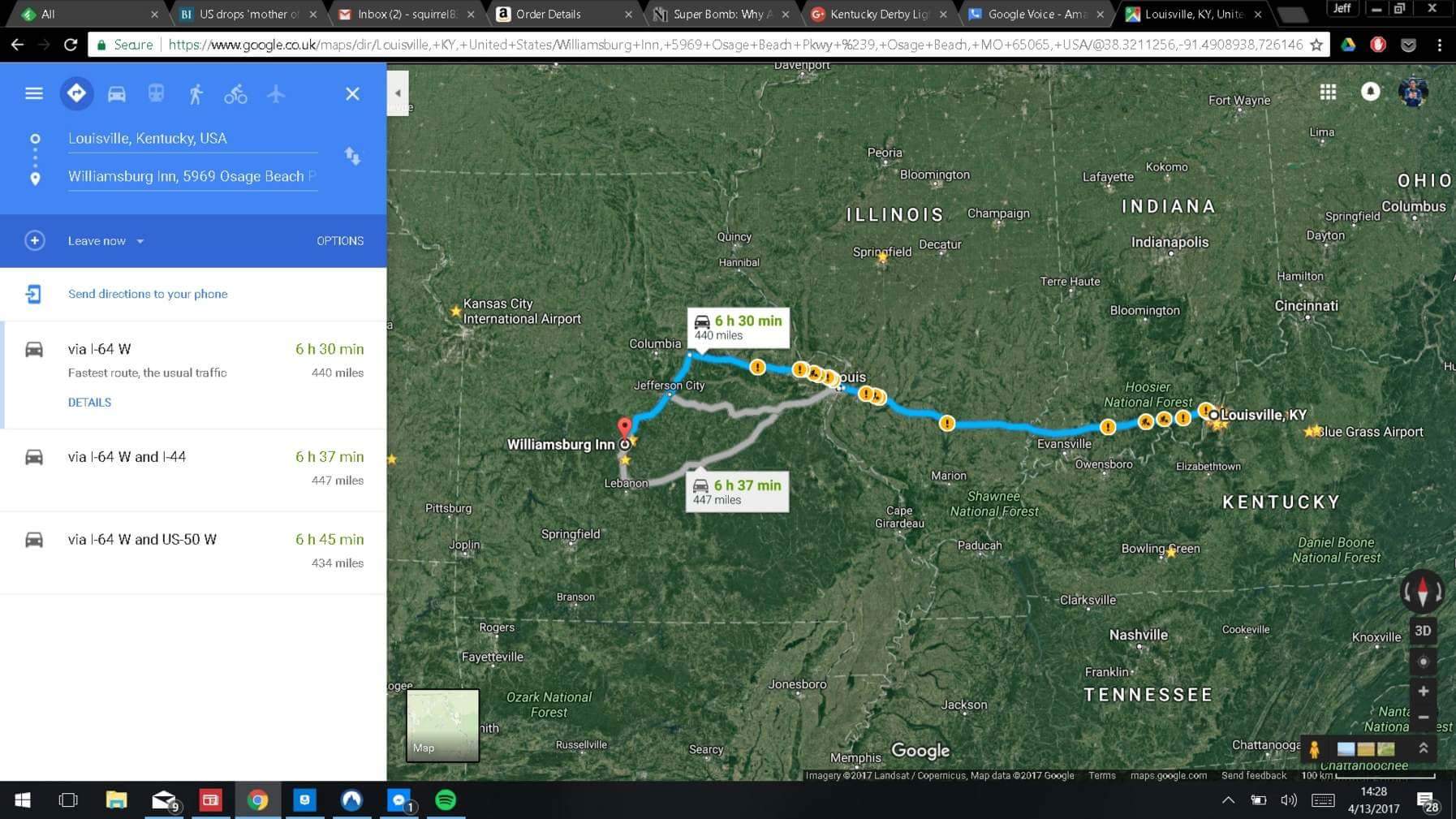This is a horizontally rectangular image, a screenshot taken from a computer monitor displaying a browser window with multiple tabs open. The top of the screen shows a black tab bar with various tabs, including "A, All," "U.S. Drop Smother," "Inbox 2," "Amazon Order Details," "Super Bomb," and "Kentucky Derby." Just below the tab bar is the site address line. On the left-hand side of the screen, there's a blue rectangular area for inputting the current location and destination addresses, with the verbiage being somewhat blurred. Below this, a white section lists various steps required to reach the destination. The main section of the image is dominated by a green aerial view of a map, traversed by a turquoise blue path indicating the travel route. This route spans multiple states including Illinois, Indiana, Ohio, Kentucky, and Tennessee, with specific locations like the Williamsburg Inn and Louisville, Kentucky highlighted. The bottom of the screen shows a border that displays open or pinned applications.